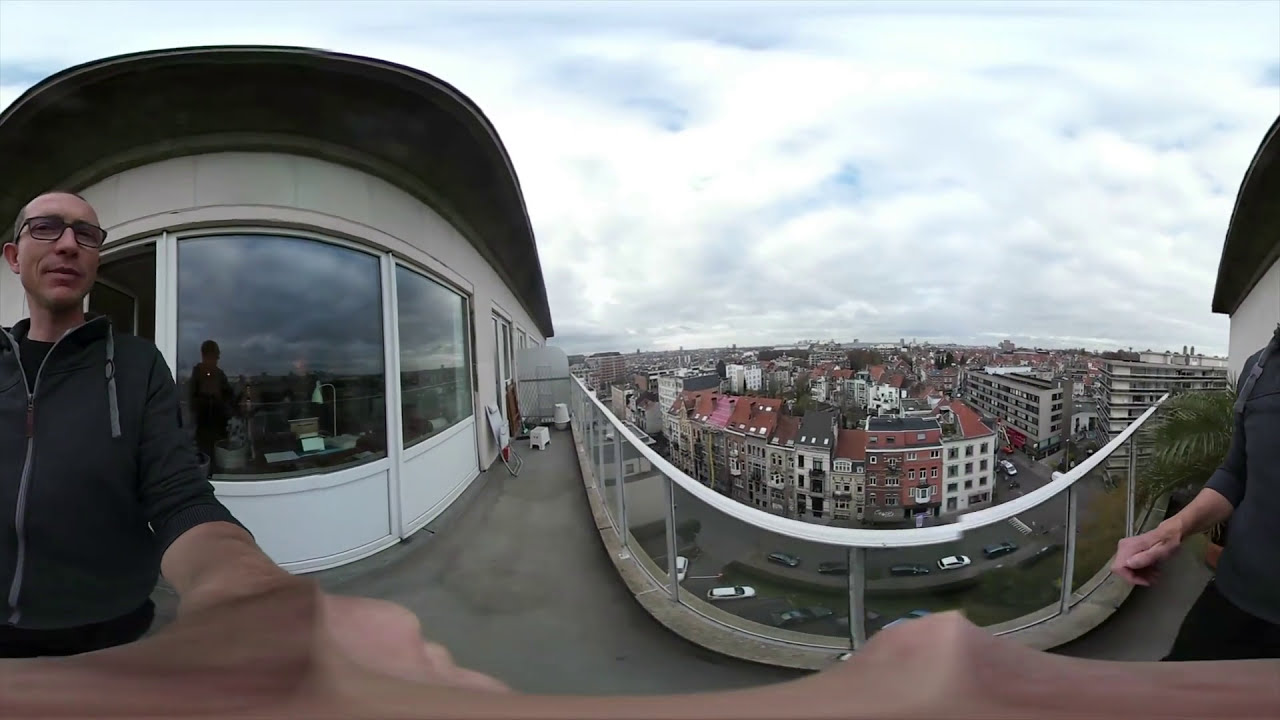In this highly detailed fisheye lens photograph, a young balding man with glasses—sporting a gray, zipped-up jacket—stands atop an observation deck that grants an expansive view of the entire city below. The observation deck itself appears to be a circular structure with large windows, a white body, and a black, hat-like roof that contrasts sharply against the cloudy sky, which has hints of blue peeking through. The city's vastness is evident from the multitude of apartment buildings, skyscrapers, government buildings, and hotels extending out into the horizon. Numerous cars can be seen parking and driving along the highways and streets below, although individual people are not discernible due to the elevated vantage point. The curved cement walkway of the observation deck guides the viewer’s eye through the image. The man’s presence on the left-hand side of the photo is also mirrored in the reflective windows of the observation building, adding depth to this dynamic urban panorama.